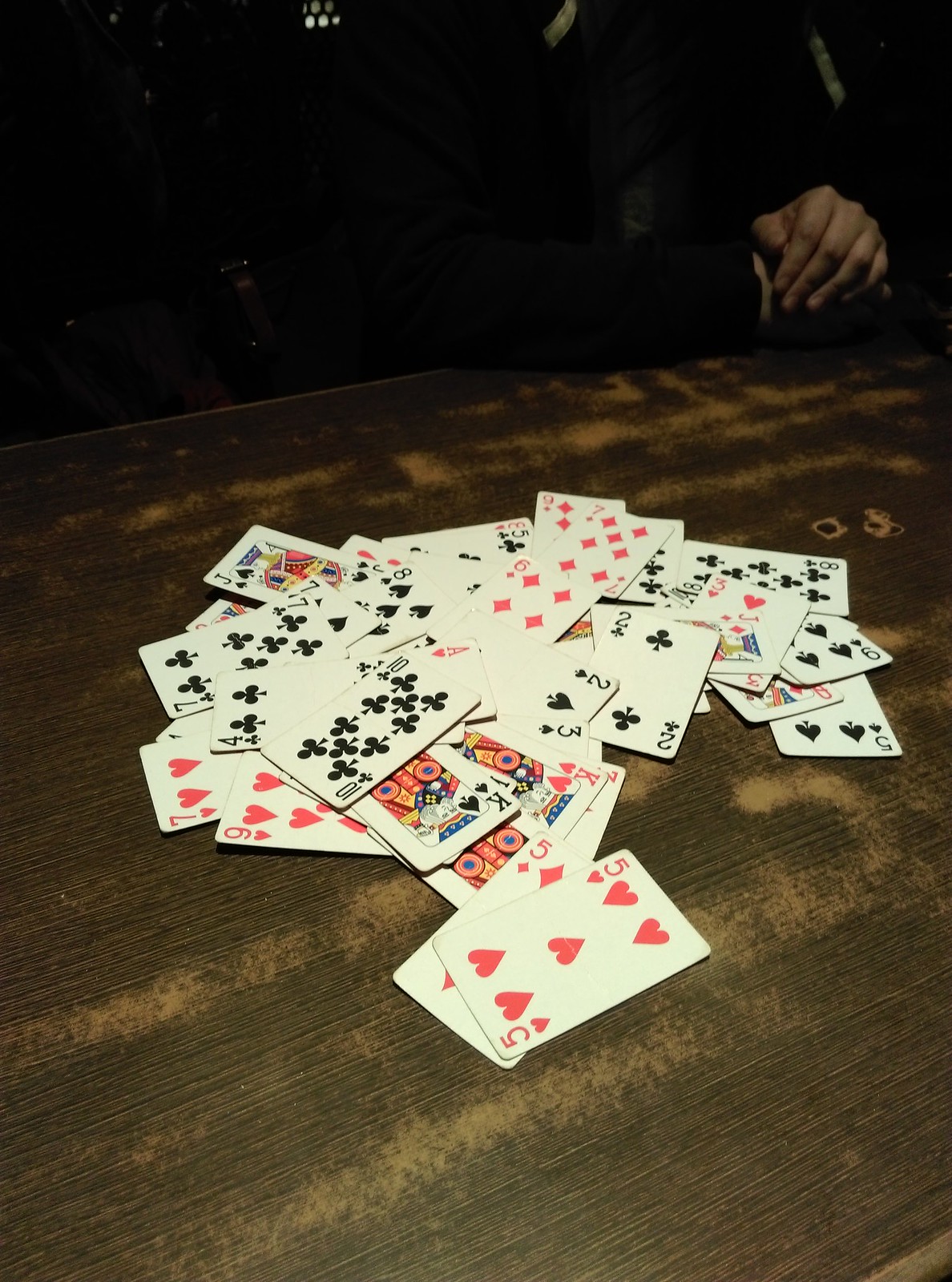In the foreground of the image, there's a detailed arrangement of playing cards spread out on a table. The cards display various suits and ranks, including numbers, King, Queen, Jack, Joker, and Ace. The table surface has visible wear marks, suggesting it is a laminate material frequently used, likely showing signs of where people's arms have rested over time.

In the upper right-hand corner of the image, a person's arm is partially visible, from the top of the arm down to their hand. This individual appears to be wearing a coat, long-sleeve shirt, or pullover, though the exact garment is indistinguishable. To the left of this person, there's an empty chair, indicating a potential empty seat at the table.

The table itself has a varied color scheme, featuring shades of brown, light brown, cream, and green. The green area of the table extends from the bottom up towards the upper right, blending into the laminate surface. Scattered across the table, the cards appear clean and well-maintained, with only the faces showing the suit and rank visible, rather than the decorative backs. The deck seems to be either full or nearly complete, comprised of many cards piled together.